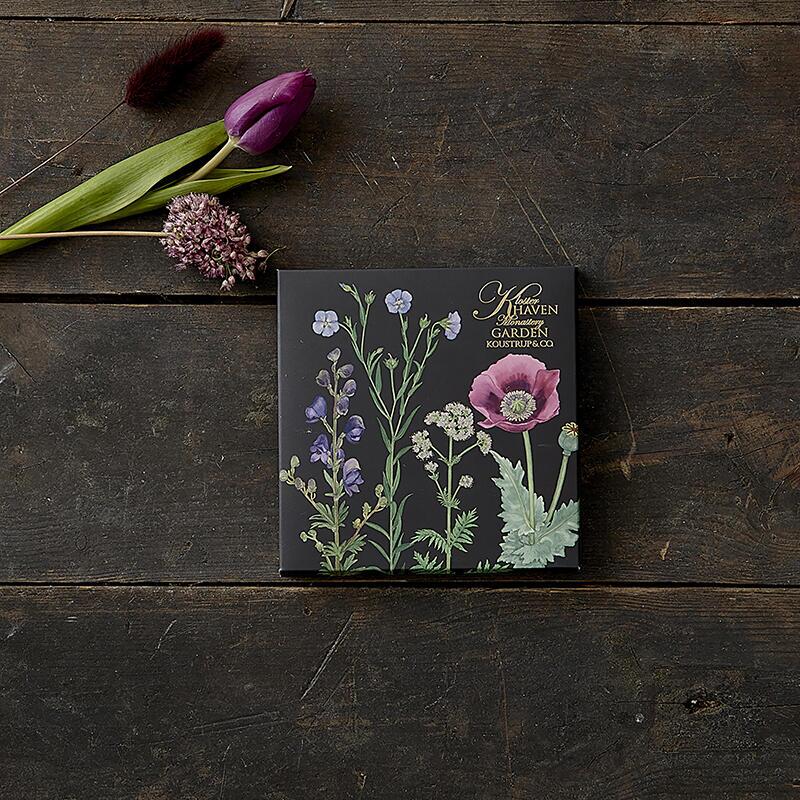This detailed photograph showcases a black square box resting on a rustic, dark mahogany wooden plank floor. The image is captured from an aerial perspective, allowing for a clear, straight-down view. The floor consists of three full horizontal planks and a partial fourth plank at the top of the image, enhancing the stylish and rustic aesthetic.

In the center of the photograph, the black box features an intricate design of various flowers, each with long green stems and delicate leaves, painted against the stark black background. The flowers include light blue ones in the center, bluebells on the left, small white flowers resembling Queen Anne's Lace to the right, and a reddish-purplish poppy on the far right. In the upper right corner of the box, there is gold text that reads "Kloster Haven Monastery Garden, Kostrup & Co."

Additionally, the upper left corner of the box displays three floral stalks: a brown, brush-like Indian paintbrush or wampus grass at the top, a purple tulip in the middle, and a flower with light pink-purple buds at the bottom. This intricate packaging against the dark wood surface combined with the detailed florals and elegant gold lettering makes for a sophisticated and visually appealing composition.